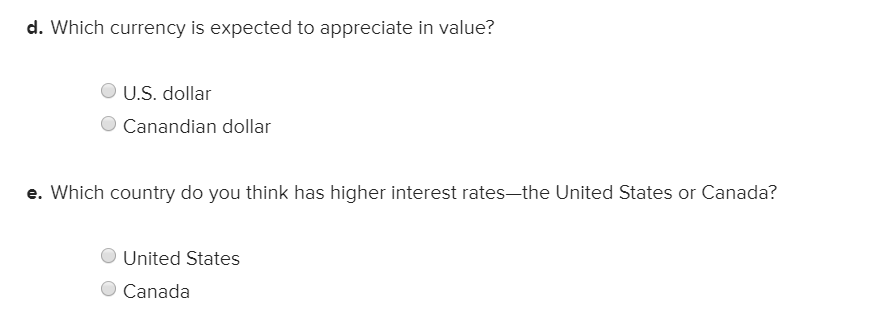This image showcases a minimalist multiple-choice test page with two distinct questions. The first question is located at the top left of the page and is labeled "D." in bold, lowercase text. It asks, "Which currency is expected to appreciate in value?" Below this question, there are two options: "US dollar" and "Canadian dollar," both accompanied by empty bubbles, indicating that no answers have been chosen. Moving down, the second question is marked with a bold "E.". It inquires, "Which country do you think has the higher interest rates?" followed by a dash and the options "United States" or "Canada." Similarly, these options are presented with unmarked bubbles. The entire page is set against a stark white background with black text, presenting a very clean, academic appearance with no additional graphics or elements. The format is clearly structured for a test or quiz, emphasizing simplicity and clarity in its layout.